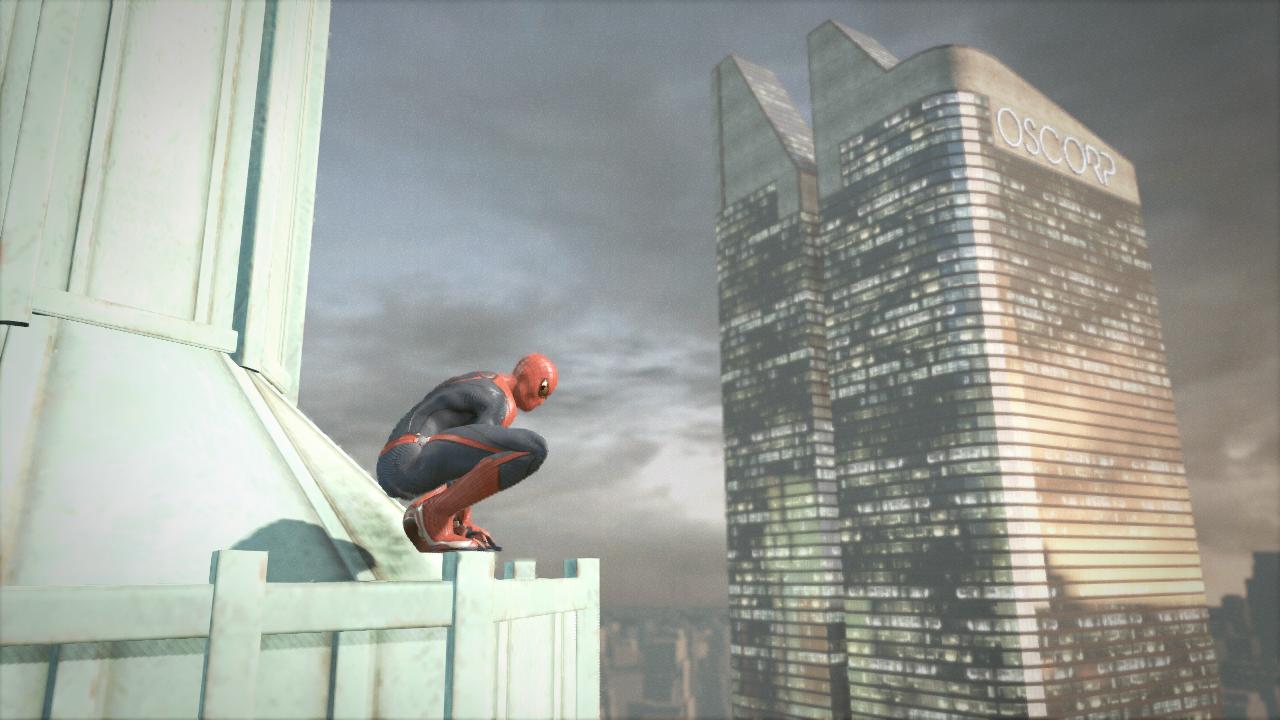In this digital illustration, Spider-Man is captured in a classic crouching pose on the edge of a tall, pale green building, set against the backdrop of an evening sky. The urban scene features another striking skyscraper across from Spider-Man, adorned with numerous illuminated windows that outline the structure. At the pinnacle of this twin-towered office building, the letters "O-S-C-O-R-P" are prominently lit, indicating the infamous Oscorp Headquarters. The twin towers rise majestically, tapering into sharp points, adding to the dramatic skyline of the bustling city.